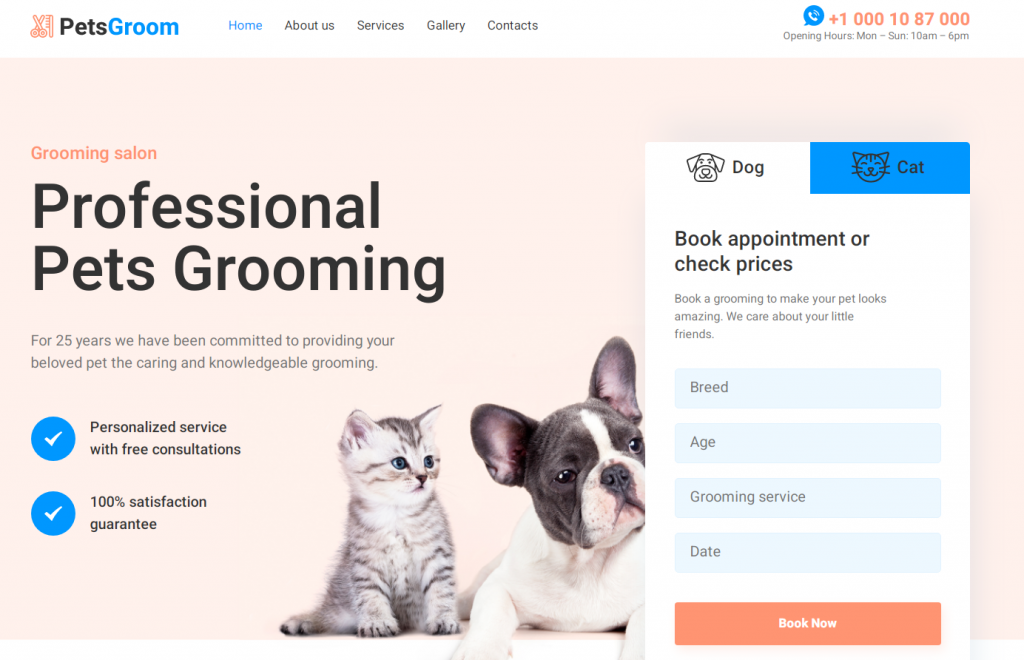The image showcases an advertisement for "Pets Groom," a professional pet grooming salon. The brand name "Pets" is highlighted in black, while "Groom" is in blue. On the left side of the image, there are red-outlined icons of a pair of scissors and what appears to be a comb. Next to the "Pets Groom" logo is a navigation menu featuring "Home" in blue, and "About Us," "Service," "Gallery," and "Contacts" in black.

On the right side of the image, there is a phone icon followed by the contact number +1 000-108-7000. The opening hours are listed as Monday through Sunday, from 10 a.m. to 6 p.m. Further text on the left side reads "Grooming Salon Professional Group Pet Grooming," emphasizing their 25 years of commitment to providing knowledgeable and caring pet grooming services.

Two blue circles with white check marks highlight key features: "Personalized services with free consultations" and a "100% satisfaction guarantee." The central part of the image features a photograph of a kitten and a small French Bulldog.

Below the photograph, tabs for "Dog" and "Cat" categories are displayed, with the "Cat" tab currently highlighted in blue and the "Dog" tab in white. Underneath these tabs are options to "Book Appointments" or "Check Prices" with a note stating, "Book a grooming to make your pets look amazing. We care about your little friend."

A form section contains data fields for "Breed," "Age," "Grooming Services," and "Date." The "Book Now" button is prominently displayed in orange with white font. The data fields are colored in shades of blue, with black font for the text.